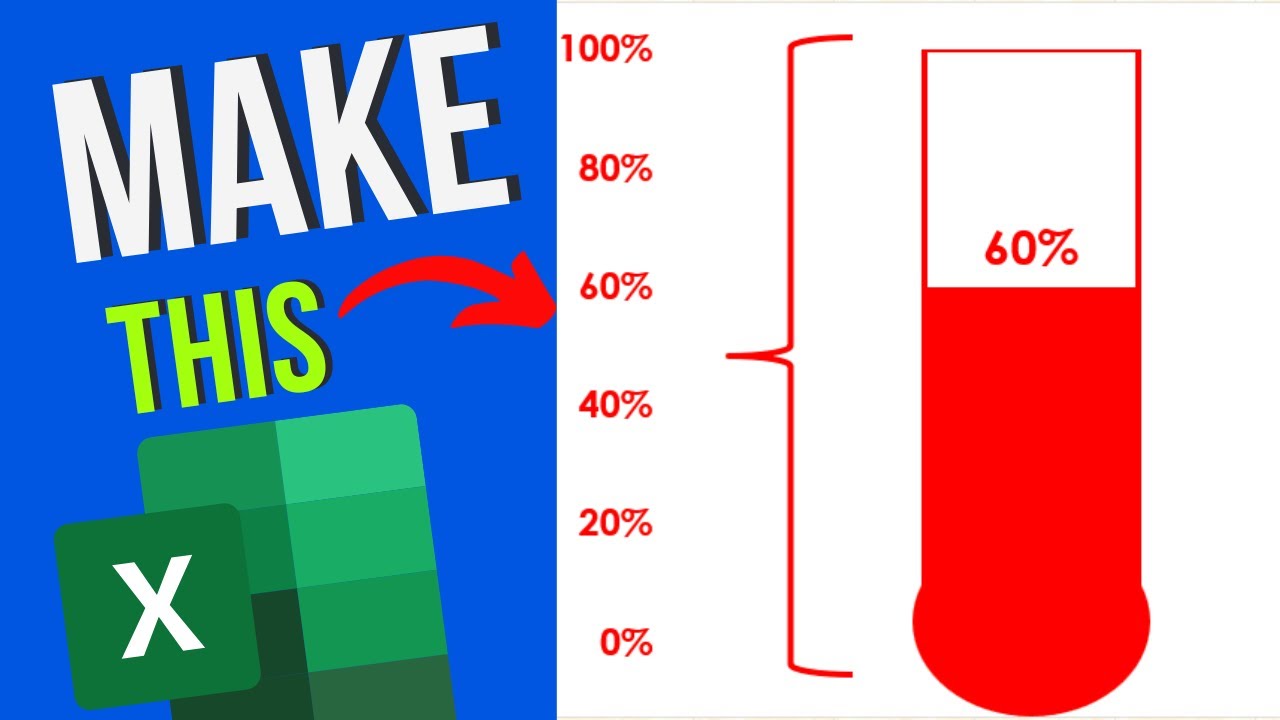The YouTube thumbnail for a Microsoft Excel tutorial features a bold and attention-grabbing design. On the left side, set against a blue background, large white text reads "MAKE" followed by "THIS" in green. Below this text, a vibrant red arrow points to the right, directing viewers' attention to the tutorial's main focus. At the bottom left, the recognizable green Microsoft Excel logo, consisting of a white "X" on a green square with a shaded green rectangle backdrop, is prominently displayed. The right side of the image features a detailed graphical element: a white square with vertical percentage markers ranging from 0% to 100%. A large, bracket-like element encompasses a vial or thermometer that is visually filled with red color up to the 60% mark, denoting the progress or value being discussed. Above this mark is a numerical "60%", reinforcing the measurement visually indicated by the thermometer. This clear and visually engaging thumbnail effectively conveys the tutorial's subject: creating a graph or progress indicator in Microsoft Excel.